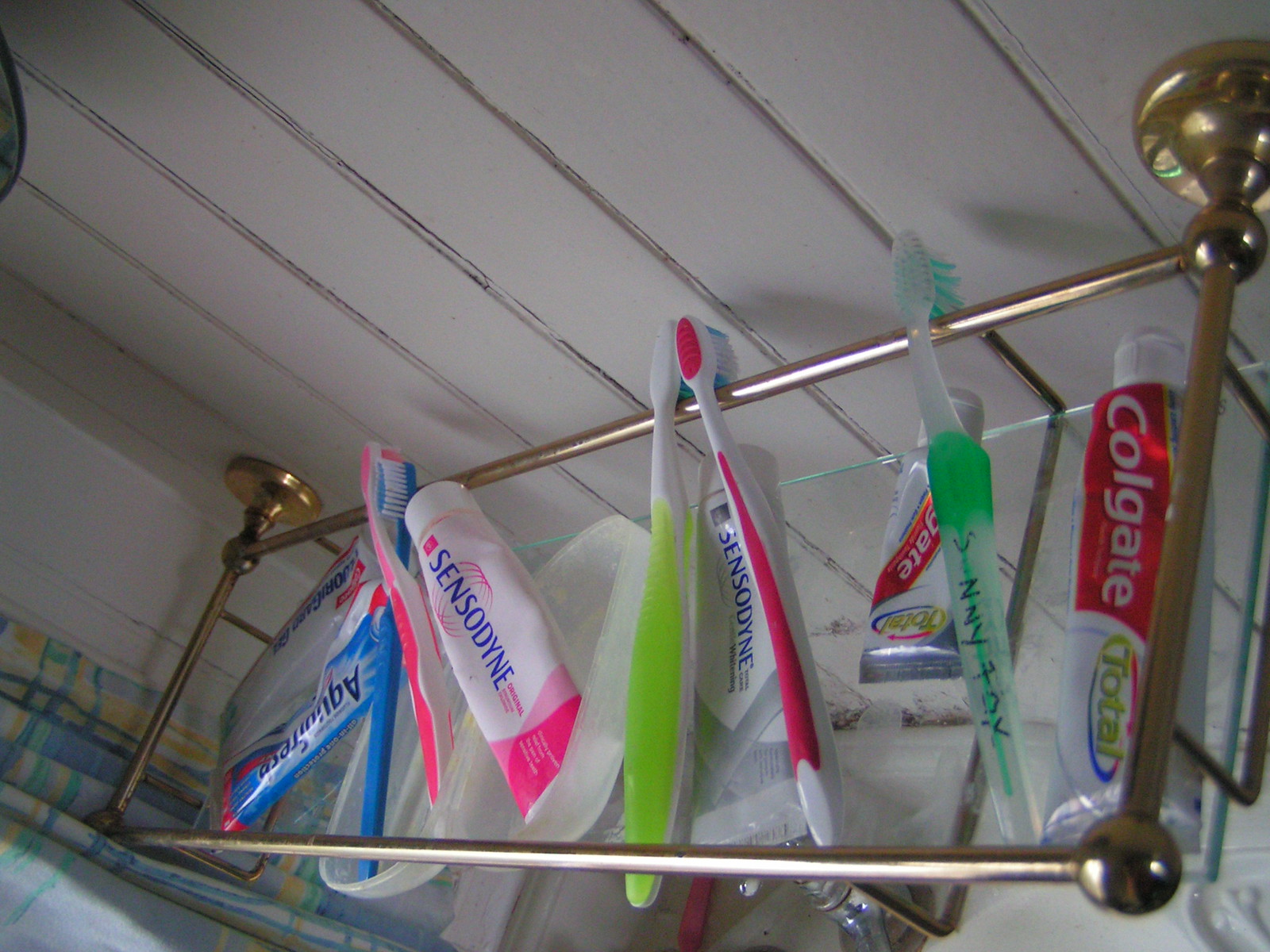This detailed color photograph depicts a gold bathroom shelf with a glass bottom, mounted on a white-painted wooden wall with vertical planks, resembling wainscoting. The photograph appears to be taken at an unusual angle, possibly tilted or upside down, adding a quirky aesthetic to the composition. To the left of the shelf, a multicolored curtain featuring shades of blue, green, yellow, and white hangs, suggesting the presence of a window.

On the gold shelf, a collection of six toothbrushes and six tubes of toothpaste are neatly arranged. The toothbrushes come in a vibrant array of colors: a green one with an inscription, a red one, a neon yellow one, a pink and white one, and a turquoise one. The toothpaste assortment includes two Colgate tubes, one larger and one smaller, two Sensodyne tubes in white and pink, an Aquafresh tube in bluish packaging, and another unidentified tube. Each toothbrush seems to correspond with a tube of toothpaste, indicating a personalized setup for multiple users. The overall image conveys an organized yet lived-in bathroom space with a hint of individuality and color.